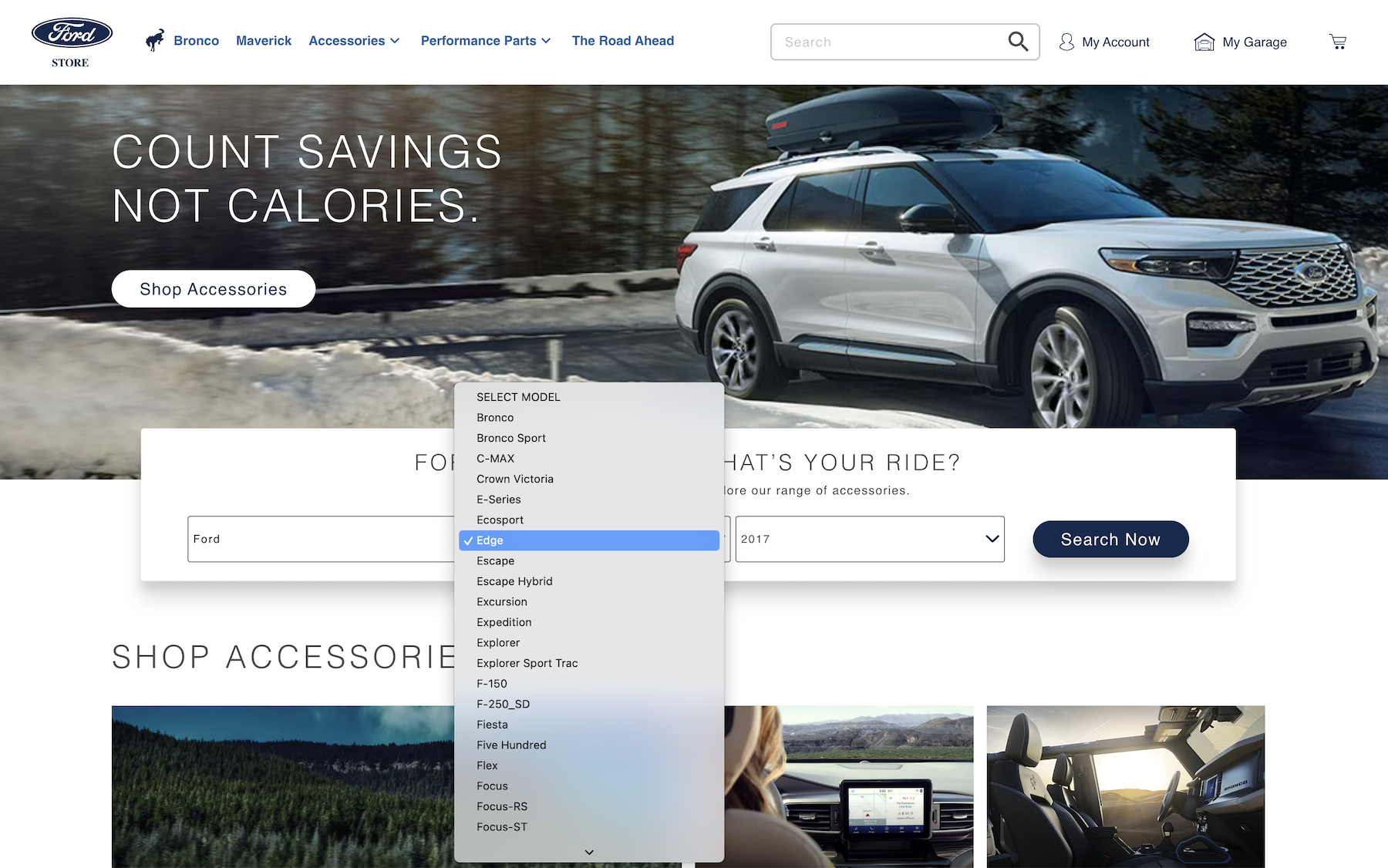This image, sourced from a Ford automobile dealer's website, prominently features a white-silver SUV with a luggage carrier affixed to its roof rack. Set against a rugged wilderness backdrop, the SUV is depicted near a rocky terrain and what appears to be a fishing dock in the background. The webpage includes sections with clickable options, one of which is a prominently displayed dropdown menu labeled "Select Model." The menu lists various Ford vehicle models alphabetically, starting with Bronco, Bronco Sport, C-Max, Crown Victoria, E-Series, EcoSport, and Edge. A checkmark marks the selection of a model in blue. The dropdown menu continues with additional models such as Escape, Escape Hybrid, Excursion, Expedition, and Explorer, extending down to the models starting with F.